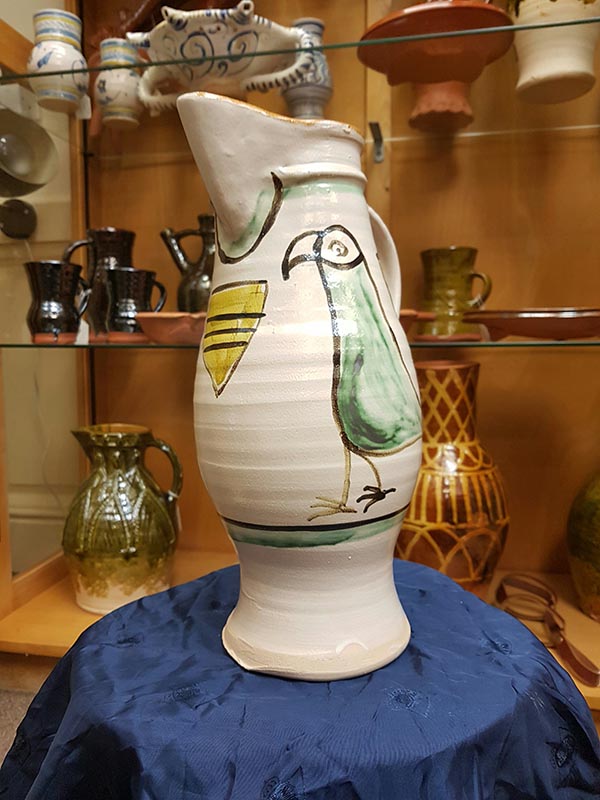The photograph captures a cream-colored ceramic pitcher, prominently displayed on a stool draped with a blue blanket. The pitcher, possibly of historical significance, showcases a simplistic and somewhat amateurish green bird painted on its surface, with brown stick-figure legs and a toucan-like curved beak. Additionally, the pitcher features a yellow triangle adorned with black stripes and green and black striping around its circumference. The pitcher is part of a larger collection, evident from the glass case filled with various ceramics and pottery pieces in the background. The setting, which hints at a museum display, emphasizes the rustic, handmade nature of the focal pitcher, likely intended for catalog-style presentation.